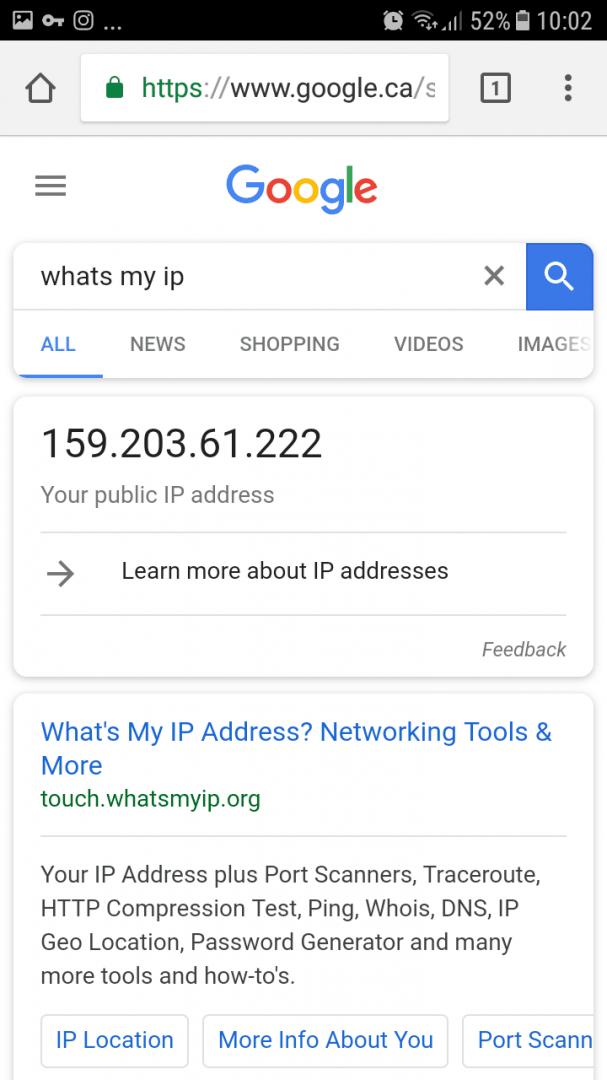The image is a screenshot of a smartphone displaying a web page. At the very top of the screen, there's a familiar black bar featuring standard cell phone icons. Below this bar, a search bar is prominently displayed, along with the usual colorful Google logo. Within the search bar, the text "what's my IP" is entered.

Directly beneath this search input, several tabs are listed: All, News, Shopping, Videos, and Images. Below these options, within a prominent box, is the information regarding the user's public IP address, which is displayed as "159.203.61.222." 

Accompanying this IP address, there's a gray bar that invites users to "Learn more about IP addresses," and another gray bar at the top right corner, marked "Feedback."

Further down, a blue box is visible with the bold text "What's My IP Address? Networking Tools and More," accompanied by a green link, "touch.whatsmyip.org." 

Beneath this section, there's an extensive list of tools and tests available, including "Your IP Address," "Port Scanners," "Traceroute," "HTTP Compression Test," "Ping," "Whois," "DNS," "IP Geolocation," "Password Generator," and many more instructional resources.

Finally, towards the bottom of the image, there are three distinct white boxes with blue lettering from left to right: "IP Location," "More Info About You," and "Port Scanner," detailing additional features and tools available on the web page.